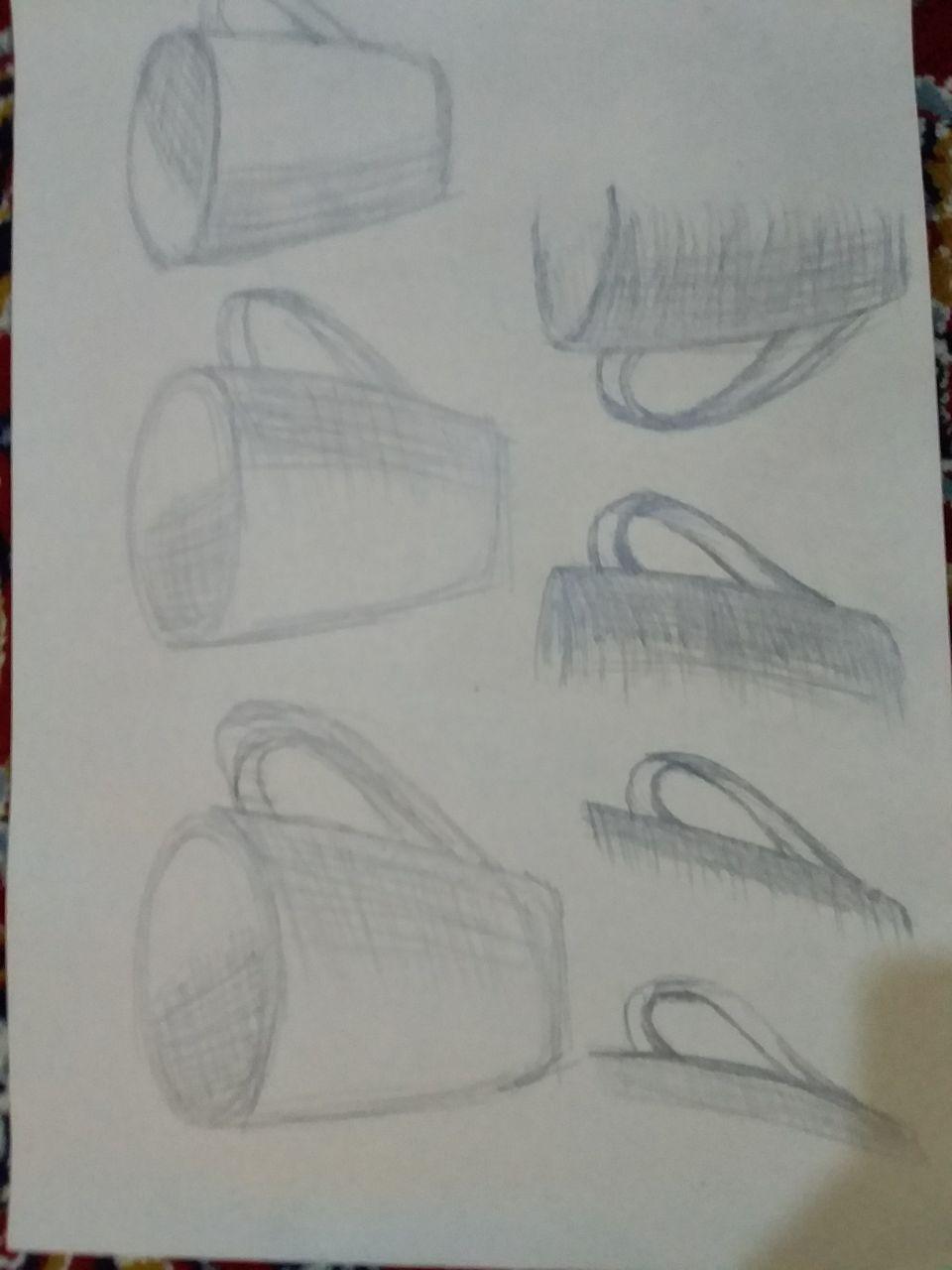This detailed pencil drawing, executed in monochromatic tones, showcases a series of white mugs meticulously arranged in two rows. In the first row, three white mugs are depicted sequentially from left to right, with the first mug being slightly larger than the second, and the third being the smallest. Each mug features a prominent handle. 

In the second row, the drawings focus closely on the handles of the mugs:
1. The first image shows just the handle with a fragment of the mug.
2. The second image highlights the handle with a slightly larger portion of the mug.
3. The third image captures approximately half of the mug along with its handle.
4. The fourth image also shows half of the mug and its handle but positioned in a different direction compared to the previous three.

The detailed rendering of each element, particularly the handles, showcases the artist's skill in capturing both the form and subtle variations of the objects.